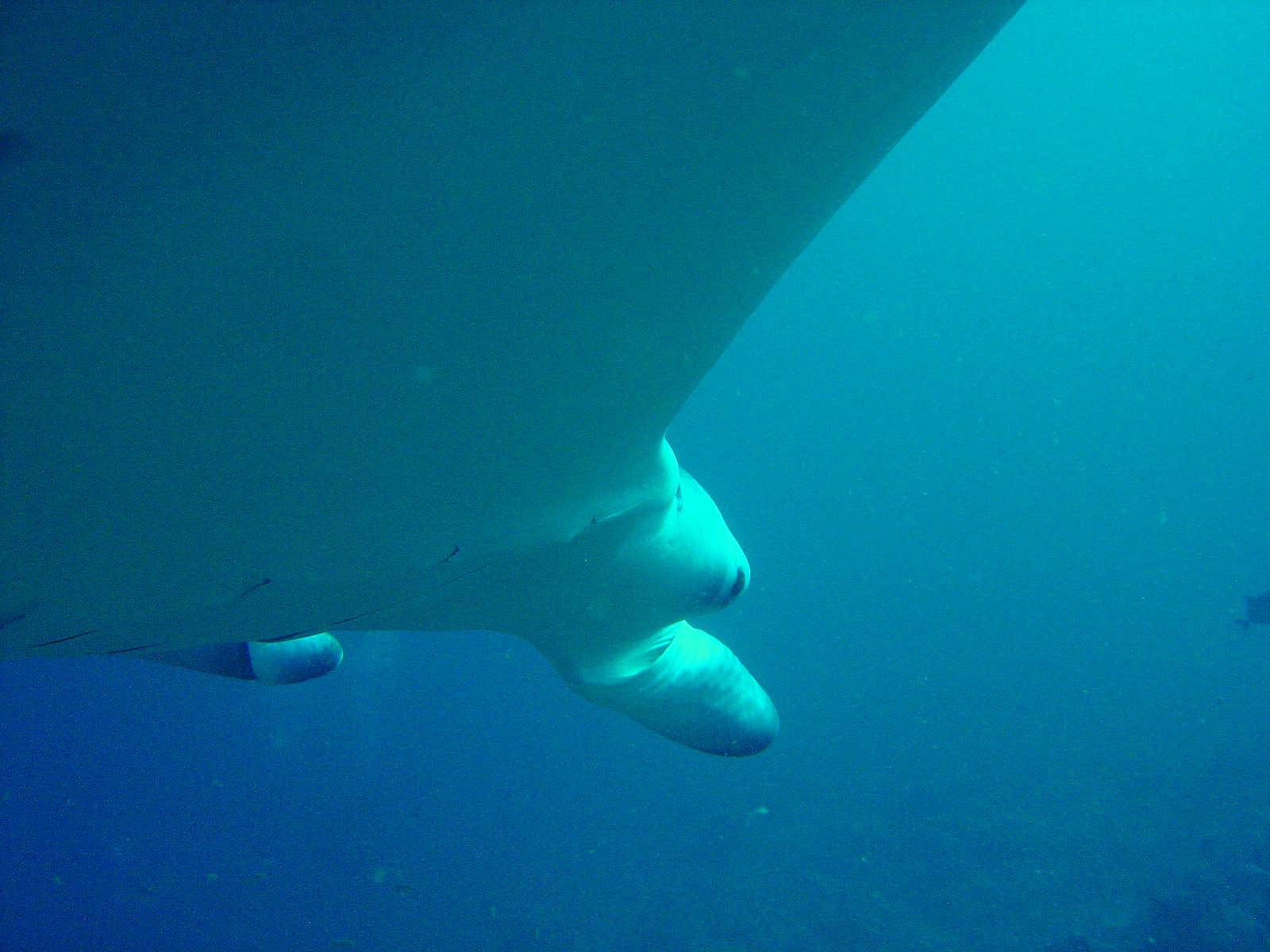This underwater image predominantly features varying shades of blue, creating a captivating and somewhat enigmatic scene. The top half of the picture is dominated by the underside of an abstract, predominantly white shape that could be interpreted as the bottom of a boat, a turtle, a stingray, or even a flotation device. This surface is mostly smooth but features two nubs toward the lower center and an additional appendage protruding from the lower left corner. Shadowing is evident in the upper left corner of the image, while highlights are concentrated toward the middle to lower portions. The form has an irregular, almost organic feel, with uneven bumps resembling a piece of ginger, giving it an intriguing, ambiguous nature. The water itself appears darker at the bottom of the image and lighter toward the top, suggesting light is filtering in from above. Hints of the seafloor and possibly a distant fish add to the underwater atmosphere.